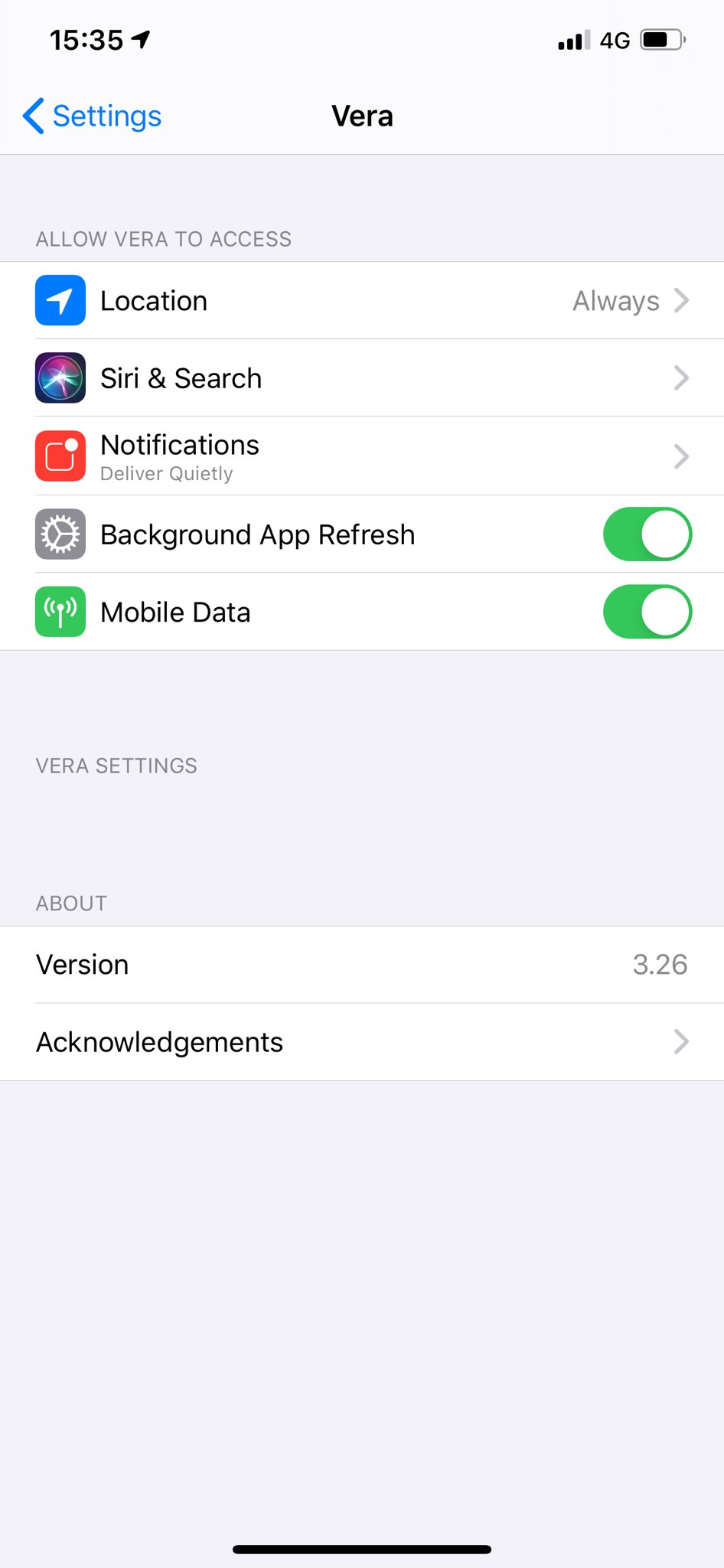The image displays the settings screen for an app named Vera on an iPhone. At the top of the screen, the current time is shown as 15:35, with the signal status indicating a 4G connection with full signal bars and the battery status visible. The title "Settings" is positioned at the top left, accompanied by a back arrow, suggesting the user is within the Vera app settings.

Below the title, the app name "Vera" is prominently displayed. Under the section titled "Allow Vera to Access," there are five permission options: "Location" (set to "Always" with a blue arrow on the right), "Siri & Search," "Notifications," "Background App Refresh," and "Mobile Data."

Further down, it lists app information under the Vera settings, which includes the version number "Version 3.26" and "Acknowledgements" with an arrow to the right that indicates additional details can be accessed by clicking.

This settings screen allows users to manage permissions and view app-related information for the Vera app. The app requests access to specific information, including constant location tracking, likely to provide location-based services.